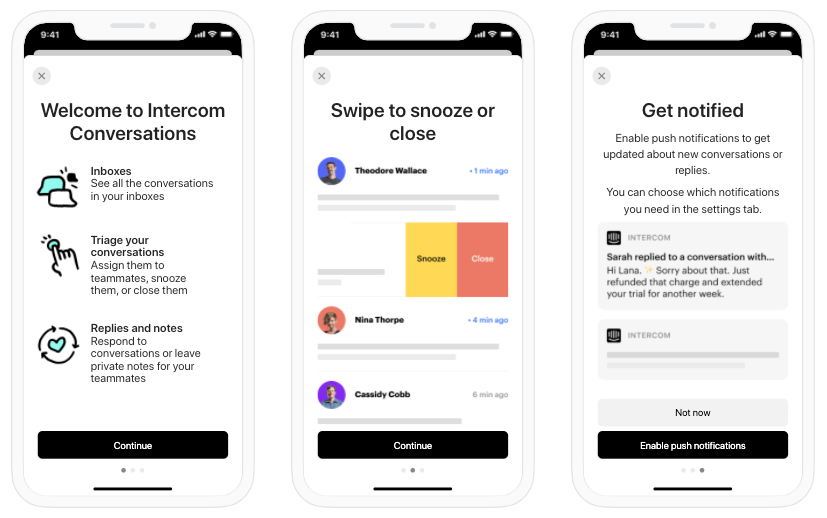The image showcases three distinct user interface (UI) layouts for a mobile application, presented side by side on a phone template. 

On the far left, the interface welcomes users with the text "Welcome to Intercom Conversations". Below this welcoming message, there are three icons: a speech bubble representing "Inboxes", a hand pressing a button signifying "Triage", and a heart surrounded by an infinite arrow cycle, indicating "Your Conversations and Replies and Notes". Each icon is accompanied by a brief description elucidating its function.

The middle interface features a header reading "Swipe to Snooze or Close". This page is adorned with graphical elements such as charts and user icons, suggesting a focus on managing or interacting with conversation metrics and user interactions.

Finally, the interface on the right displays the message "Get Notified". It invites users to enable push notifications to stay updated on new conversations or replies, additionally indicating that notification preferences can be customized within the Settings tab.

All three UI layouts maintain a minimalist design with a white background and ample empty space, ensuring a clean and uncluttered appearance.